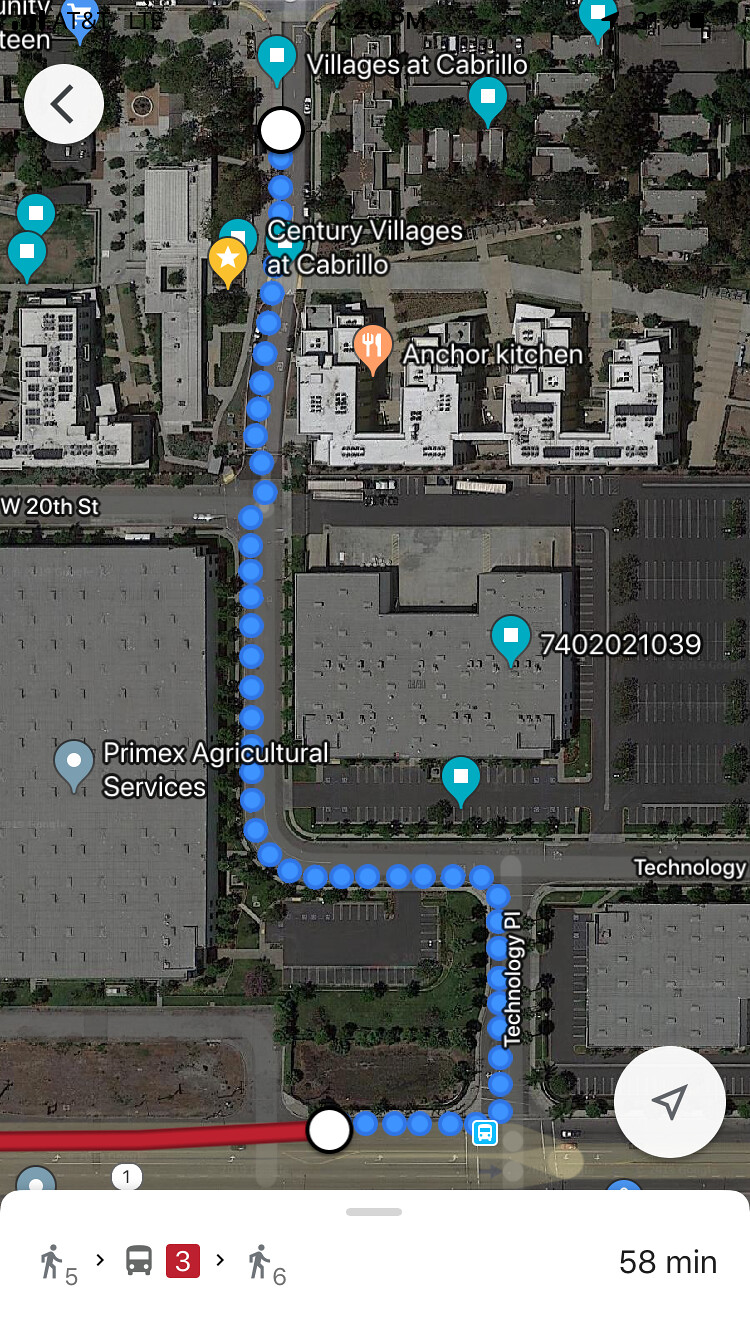This screenshot from Google Maps depicts a planned route through a mixed urban landscape. The upper section of the image highlights a residential area, characterized by a grid of streets and housing. The lower section is dominated by a large warehouse, suggesting an industrial zone. A neon blue dotted line represents the user's path, extending from the bottom of the screen to a white circular icon at the top, indicating the final destination. At the bottom right corner, "58 minutes" suggests the estimated duration of the journey. On the bottom left, an icon of a person walking, a bus icon marked with the number "3," and another walking icon illustrate the walking and public transit segments of the route. The background of this section is shaded in gray, emphasizing the step-by-step navigation instructions.